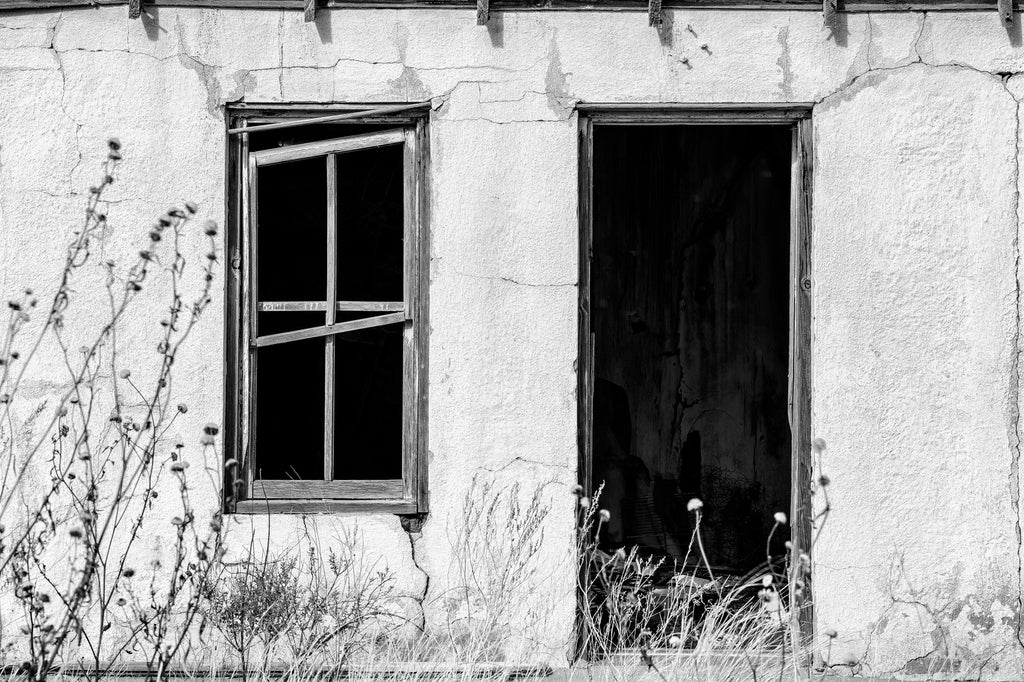This black and white photograph captures the front of an old, abandoned home made of white concrete, cracked in several places. The image is taken during the daytime and is detailed in shades of gray and black. A weathered, wooden window on the left appears broken, with some boards hanging down at an angle. An open doorway, void of a door, reveals a dark, empty interior. Above, wooden rafters are partially visible, extending slightly beyond the roofline. In front of the building, knee-high weeds and tall grass dominate the foreground, emphasizing the neglected state of the property.